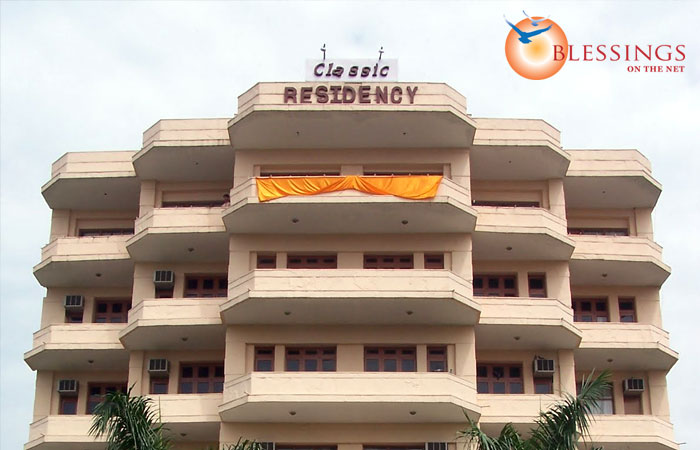The image features a multi-level building known as "Classic Residency," exemplifying an off-white or ivory-colored cement structure with built-in balconies. The photo, taken from ground level, highlights three visible floors plus the roof, with each floor extending to sections on the left and right. Most balconies house window air conditioning units. The facade of the building showcases a red sign that says "Classic Residency" on the roof, while an orange banner hangs over one balcony. 

The scene includes palm trees at the bottom left and right, suggesting a warmer climate. In the top right corner of the photo, the words "BLESSINGS ON THE NET" appear in blood orange, with "BLESSINGS" prominently capitalized. Adjacent to this text is an orange sun illustration with concentric circles in varying colors and two blue birds with white-tipped wings flying over it. The background of the image is primarily a bluish gray, possibly depicting an overcast sky.